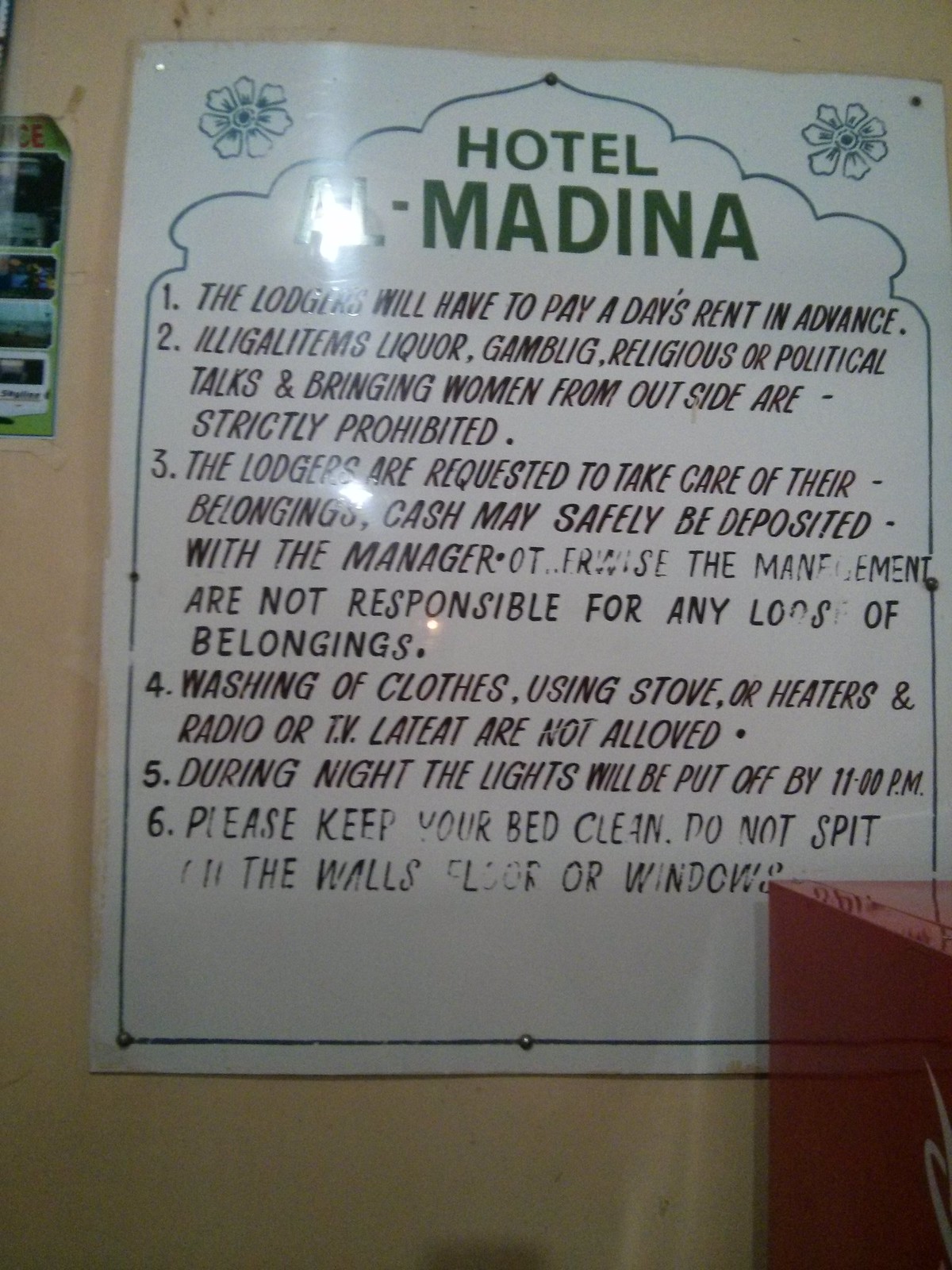A detailed white signboard, likely positioned at the entrance of a hotel, stands against a tan (or beige) wall, with a small round table situated to the bottom right of the image. The sign features the name "Hotel Medina" prominently in large green letters, with "Hotel" in smaller print above "Medina." The corners of the sign are adorned with a small green floral decoration that resembles a clover leaf. Below the hotel name, six hotel regulations are listed, with the sixth rule appearing slightly blurred, possibly written in marker and less permanent than the others.

The sign regulations read as follows:
1. The lodger must pay a day's rent in advance.
2. Illegal items, liquor, gambling, religious or political discussions, and bringing women from outside are strictly prohibited.
3. Lodgers are required to take care of their belongings, and cash may safely be deposited with the manager, as management is not responsible for any loss of belongings.
4. Washing clothes, using stoves or heaters, and operating a radio or TV late at night are not allowed.
5. Lights will be turned off by 11 p.m.
6. Lodgers should keep their beds clean and avoid spitting on the walls, floors, or windows.

The text is written in clear handwriting, although the sixth rule is somewhat difficult to read. Additionally, there is a piece of furniture, likely white with a red hue, partially covering the lower right corner of the sign, adding to the scene's detailed and structured composition.